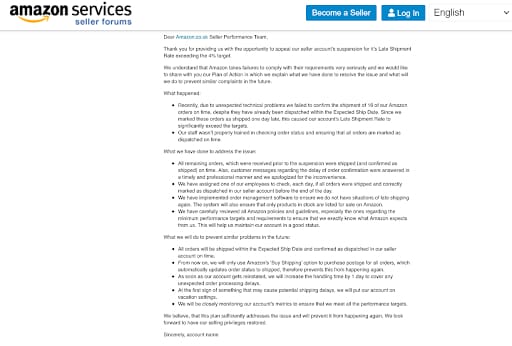This screenshot shows a web page from the Amazon Seller Forums, designed for Amazon services sellers. Dominating the top of the page is the iconic Amazon logo, alongside the 'Amazon Services' text, with options such as 'Become a Seller' displayed prominently in white lettering against a blue background. To the right, there are buttons labeled 'Log In,' also in white text on a blue background, and an icon of a small person figure, which typically signifies the user profile or account settings. Adjacent to these elements is a language selection dropdown menu, displaying 'English,' suggestive of the option to change the website's language according to user preferences.

However, the focal point of the snapshot is a partially visible message addressed to the Amazon Seller Performance Team. The readable portion begins with a polite greeting and gratitude, "Dear Amazon Seller Performance Team, thank you for providing us with this opportunity to appeal your seller account," followed by a discussion involving a "4% target." The remainder of the message is difficult to decipher due to extremely small font size, even after zooming in. The overall context suggests that this is a formal communication from Amazon services, focusing on appreciating the sellers' efforts and elaborating on their performance guidelines.